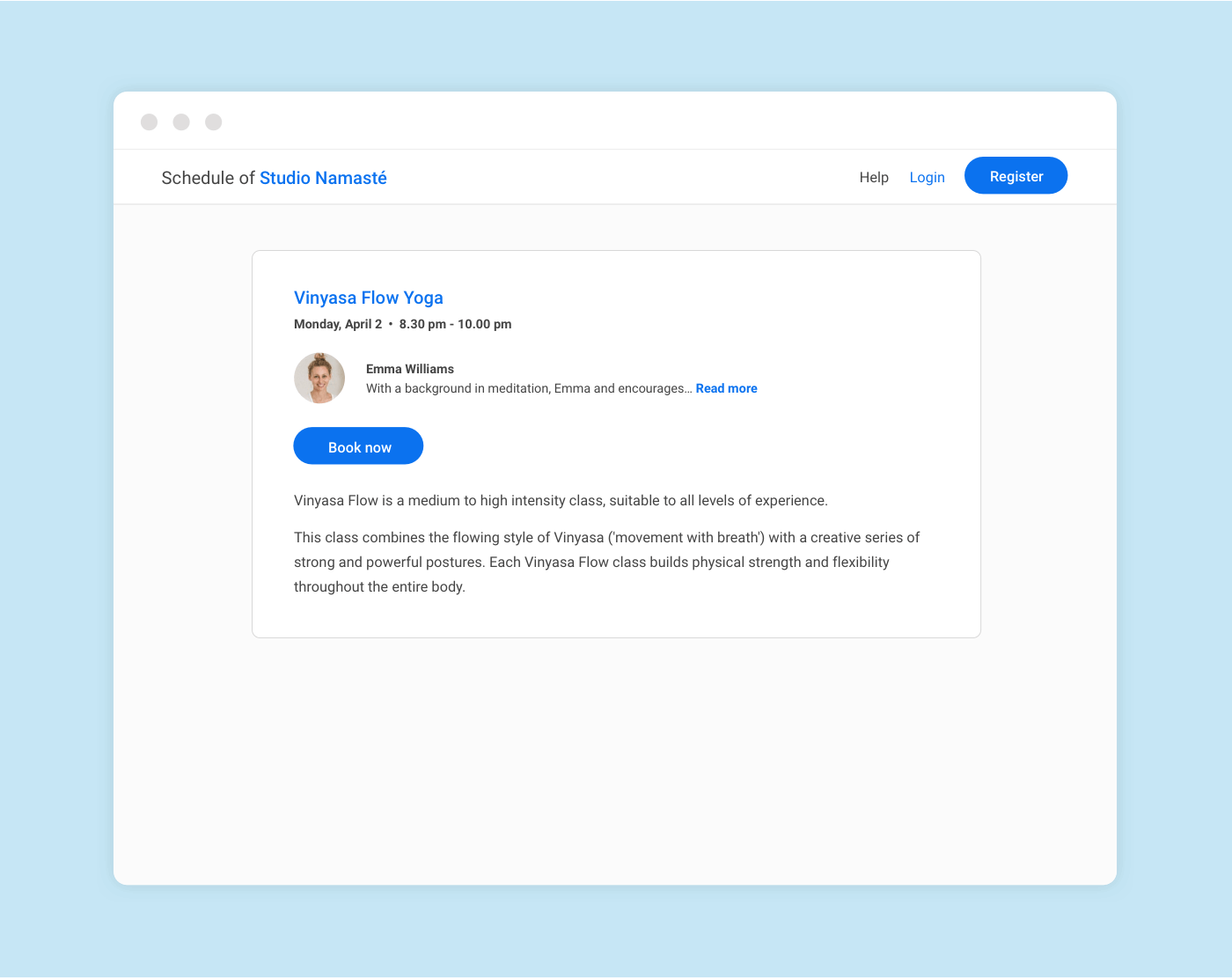**Caption**: 

The image features a light blue square with a centered white square containing detailed information. Surrounding the white square is ample negative space, accentuating its content. 

At the top of the white square, on the left, it reads "Schedule of Studio Namaste," and on the right are the options "Help," "Login," and "Register." The word "Help" is in black, "Login" is in blue, and "Register" is presented as a blue button with white text.

In the middle section, the text "Vera Stanza Flow Yoga" appears in blue. Below this, the schedule is specified as "Monday, April 2nd, 8:30 p.m. through 10:00 p.m.," followed by the name "Irma Williams." A brief description indicates that Irma has a background in meditation and encourages participants, with a "Read More" link in blue.

Further down is a "Book Now" button in blue. Below this button, a more detailed description explains that "Vera Stanza Flow Yoga" is a medium to high-intensity class suitable for all experience levels. The class combines the flow style of Vinyasa movement with breath, featuring a creative series of strong and powerful postures that build physical strength and flexibility throughout the body.

At the bottom left of the white square, there's a circular photograph of Irma Williams, a woman with blonde hair styled in a bun, wearing a white shirt.

The overall design uses blue and white colors to create a clean and inviting look.